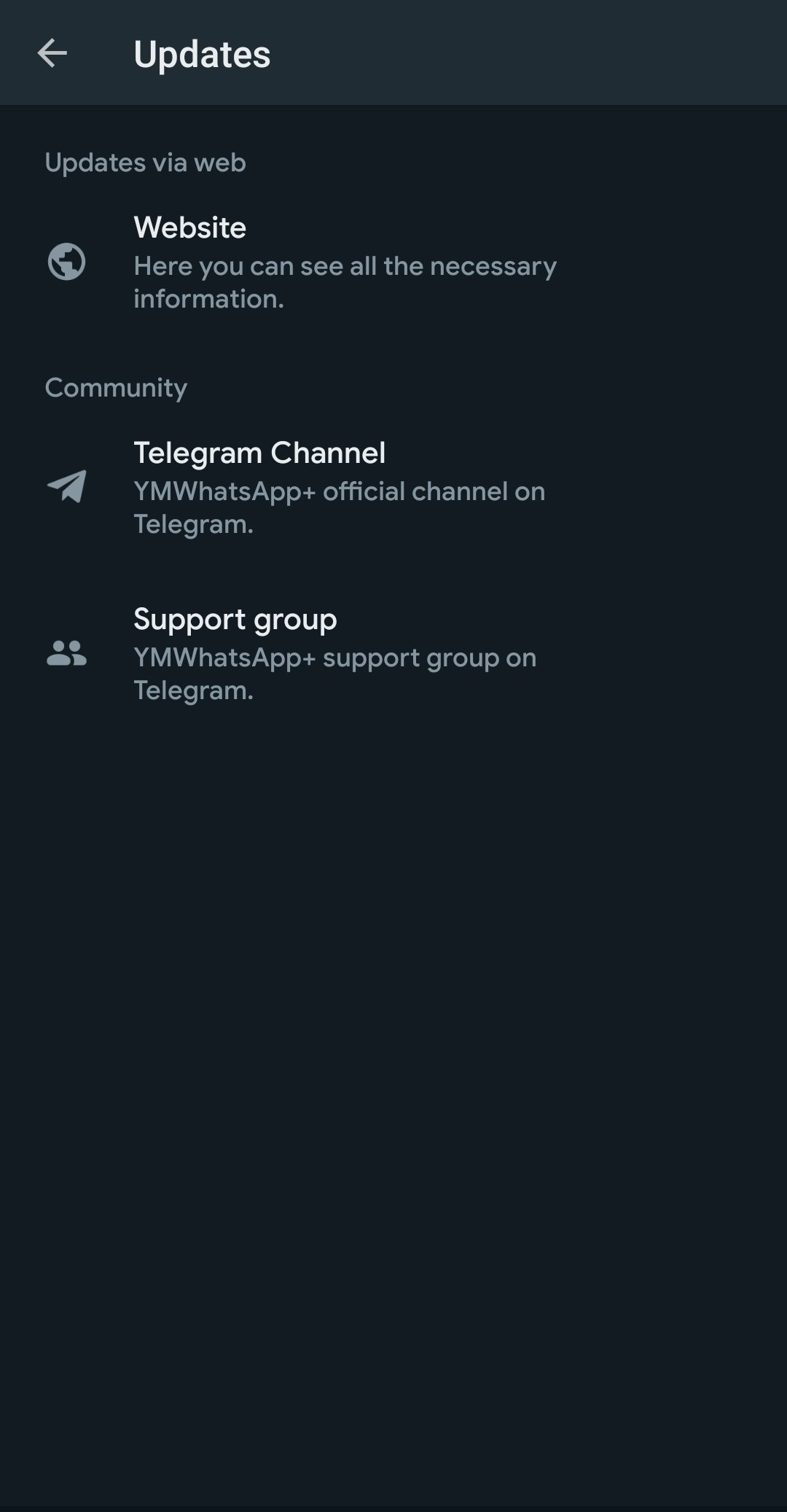The screenshot displays an updates page. At the top, there is a light grayish title bar featuring the word "Updates" in white font with a capital 'U', left-aligned. To the left of this title is a white back arrow.

Beneath the title bar, in a smaller gray font, the text reads "Updates via web." Following this section is the "Website" heading, characterized by a capital 'W' in white, paired with an earth symbol to its left. Underneath the "Website" heading, the text states, "Here you can see all the necessary information."

Next, there is a "Community" section, marked by a capital 'C' and using the same gray font color as the "Updates via web" text above. Within this section, there are references to various channels: "Telegram channel" and "WhatsApp + the official channel on Telegram."

Finally, the last section is labeled "Support Group," also in the gray font color.